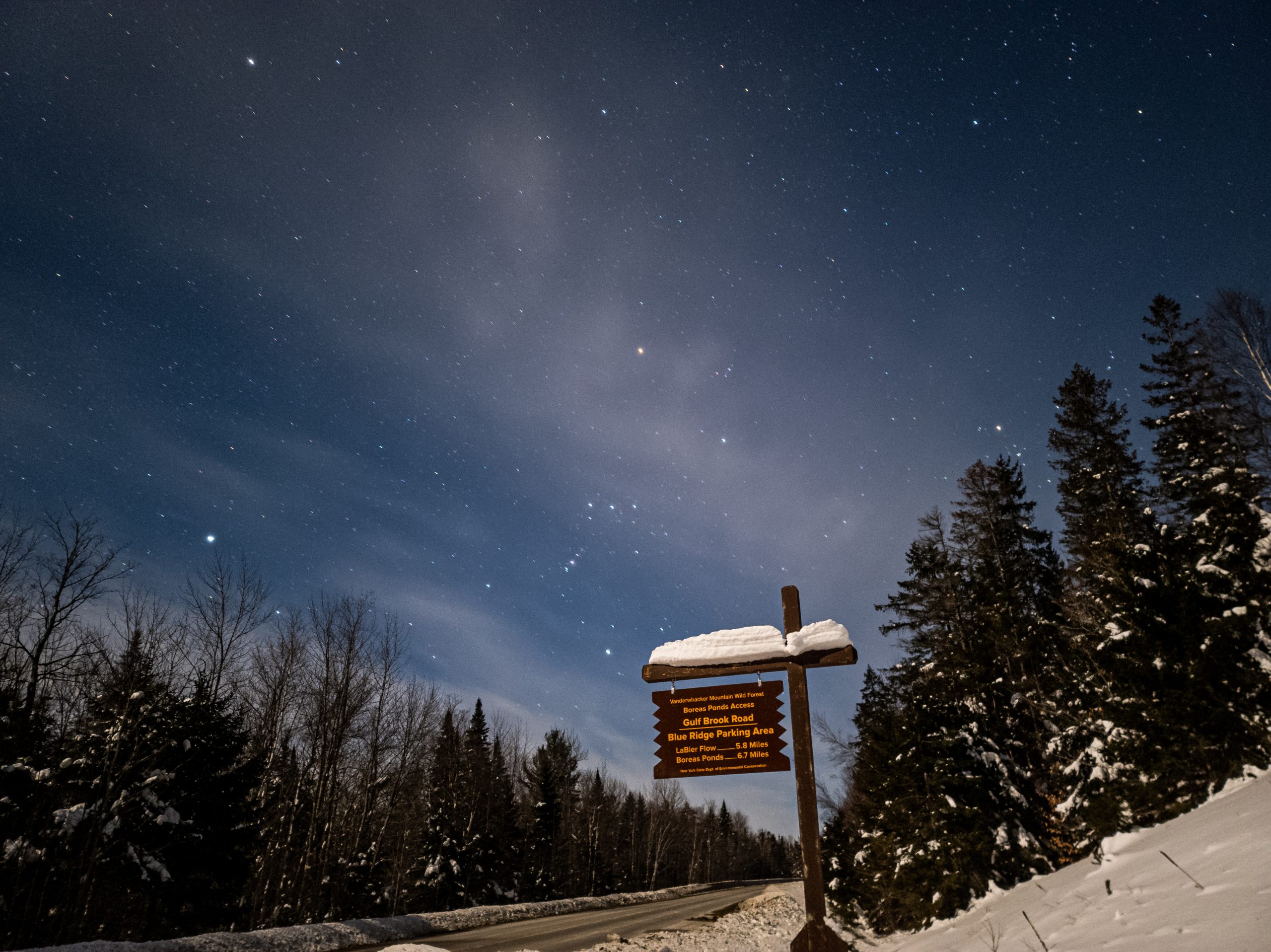In this detailed image, we observe a serene winter night scene dominated by a captivating interplay of natural and human elements. The sky above is a gradient of dark blue, almost black at the edges, speckled with what appears to be falling snow rather than stars, accentuated by hazy gray clouds. The centerpiece is a wooden road sign in the foreground, crafted from rustic beams creating a T-shape. Snow delicately piles on top of the sign, which bears yellow text that reads: "Gulfbrook Road, Blue Ridge Parking Area, LaBeer Flow 5.8 miles, Boreas Pond 6.7 miles."

This scene unfolds in a rural, snow-covered landscape with freshly plowed roads exhibiting a light layer of slush. Pine trees, their branches laden with fresh snow, line both sides of the road, creating a tunnel-like effect that draws the eye toward the horizon. Among the dense pine forest, some trees stand bare, indicating the deep winter setting. The overall ambiance is quiet and still, with no signs of vehicles or human activity, enhancing the tranquility of this snowy, rural expanse.